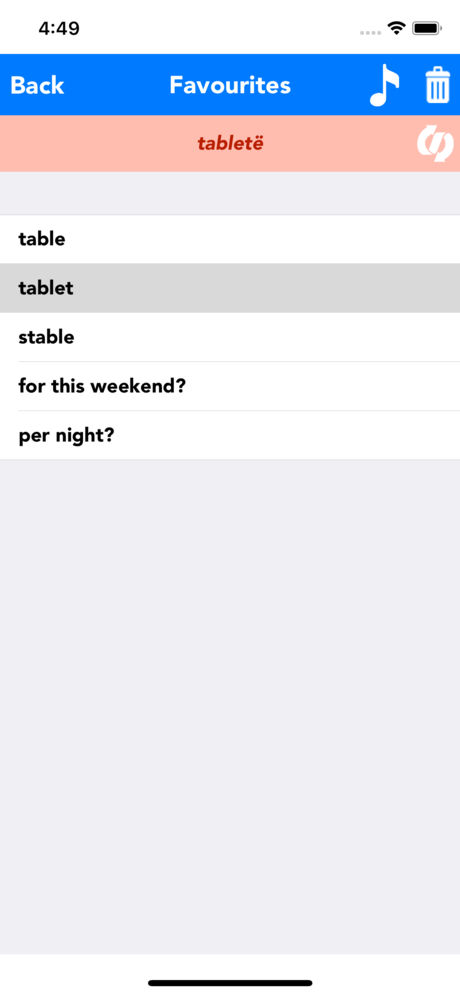This screen recording captures a screenshot taken from a phone, displaying the time as 4:49 in the top left corner. On the right side, the icons for Wi-Fi and battery life are visible. Directly below, a solid blue horizontal line spans the width of the screen. Written in white on this blue bar are the words "Back," "Favorites," a musical note icon, and a trash can icon.

Under the blue bar, there is a pink horizontal bar with red text that reads "Tablet," accompanied by a white arrow-ribbon icon. Beneath this, a gray horizontal bar follows, which is blank. 

Next, a white horizontal bar displays the word "Table." Below this, another gray horizontal bar appears with no text.

Continuing downward, another white horizontal bar states "Table," followed by a gray bar that says "Tablet." Lower on the screen, a white bar reads "Table" again. Subsequently, it says "For this weekend," followed by "One night" in a similar white bar. 

Each section is separated by a thin gray line, and at the very bottom of the screen, there is a very light gray box with a black horizontal line above it.